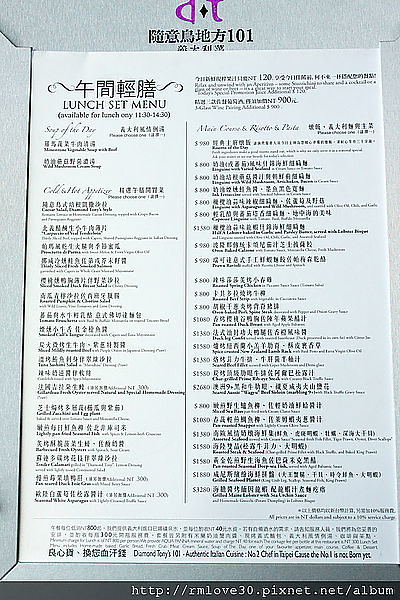The image features a lunch set menu that is predominantly white with a hint of very light blue, green, and gray hues. Positioned in the top left corner, the words "Lunch Set Menu" are clearly displayed. Despite the prominence of Asian characters throughout the menu, making it largely unreadable for those unfamiliar with the language, there are two distinct columns of menu items. The right-hand column is slightly wider than the left-hand one. While the menu items in the left column do not display prices, the right column does list prices, though the specific currency or country is indeterminate.

In fine English cursive near the top, phrases like "Soup of the Day" and "Main Courses" are visible, but the text is small and difficult to decipher. The menu rests upon what appears to be a light gray slotted menu holder, with visible lines on both sides indicating that the menu slides into the holder from the top. Just above where the menu slides in are more Asian characters along with the number 101, and a purple logo or stamp is noticeable at the menu's top.

At the very bottom of the image, there's a black band containing a URL: http://rmlove30.pixnet.net.album, which appears to be a web address for further information or possibly an album associated with the menu or the establishment.